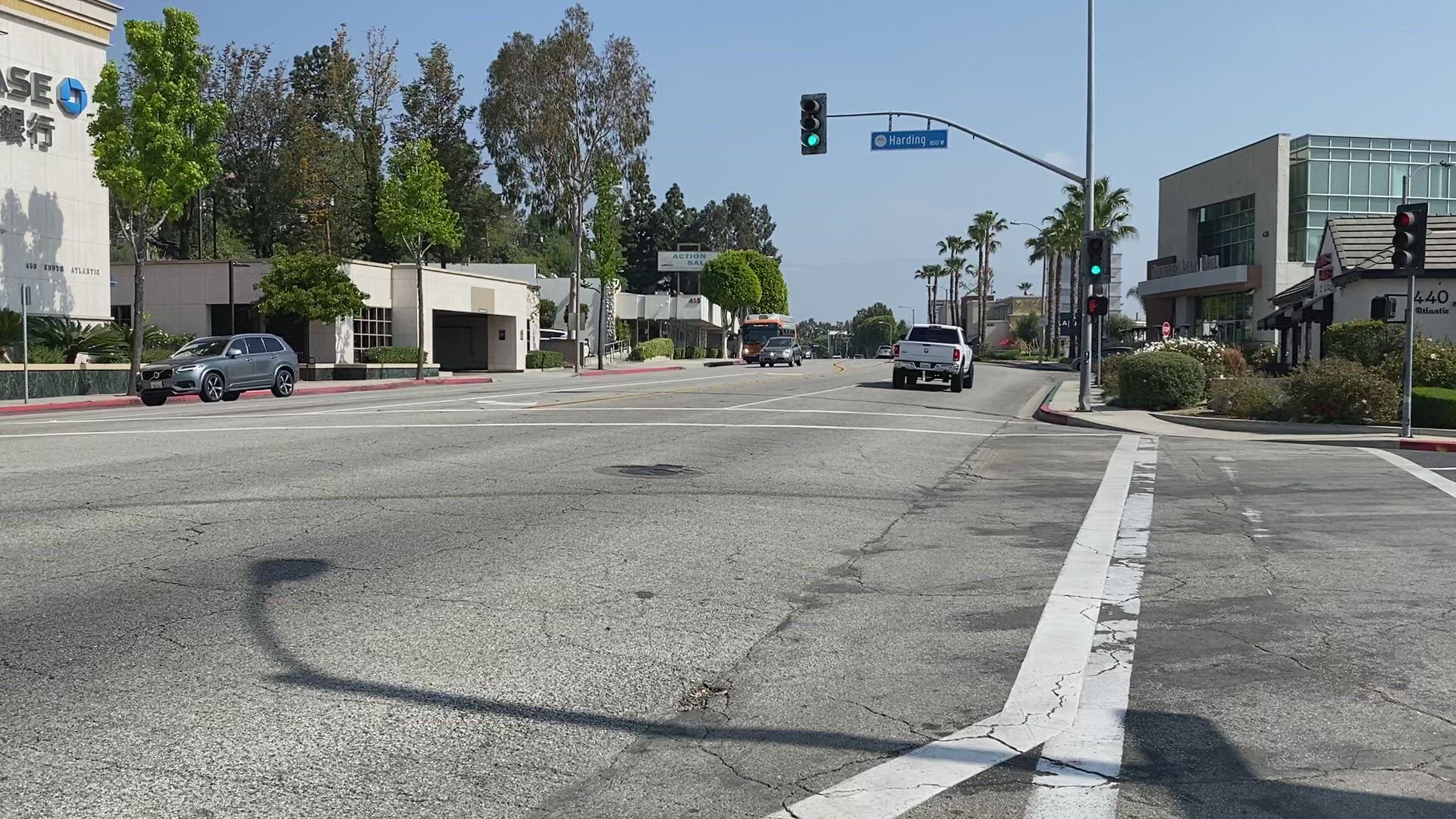The photograph is taken from the corner of a street, capturing a detailed streetscape. On the left side of the image, there's a prominent Chase Bank, easily identifiable by the visible "CHASE" logo and the partial letters "A.S.E." The building features large Chinese characters beneath the Chase name, all rendered in black against a white facade with a tan border at the top. Adjacent to the Chase Bank is a smaller, one-story white building that resembles a garage, complete with a large entrance.

The curbs on the left side of the street are painted red and run continuously down the road. A small gray SUV waits at the stoplight on this side. On the right corner of the image, there's a crosswalk, marked by white painted lines, stretching across the street.

At the bottom of the photograph, the shadow of a light pole is clearly visible on the ground. Directly ahead, a stoplight dangles from another light pole, accompanied by a blue rectangular street sign to its right. On the far right of the image, another smaller stoplight is mounted on a metal pole.

In the background, two distinctive buildings stand out. One is a smaller structure that resembles a house, marked with the number "440" on its side. The other is a taller, more modern building featuring an Art Deco style. This building boasts large glass windows at the top and a concrete archway at the front.